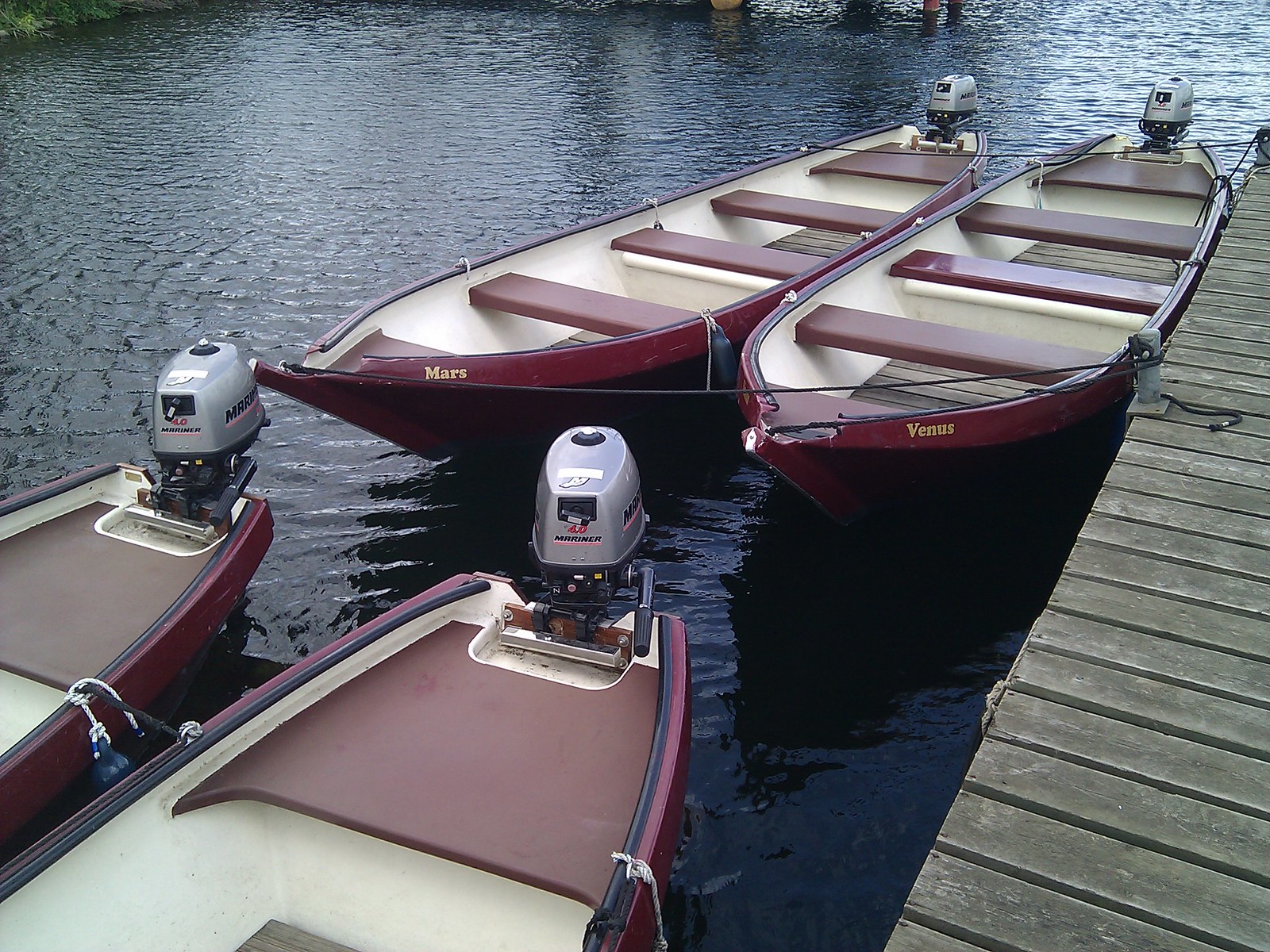This image captures a quaint scene at a weathered, brownish-gray wooden dock set against dark navy blue waters. Tied securely to the dock with long black ropes and silver hooks are four burgundy-red wooden boats, each equipped with a silver and black motor. These motors appear to be roughly 40 horsepower. The boats are open and spacious, likely seating around four to eight people. Their interiors contrast with off-white sides and brown wooden floors, made from slats of wood. Notably, the boats feature burgundy-red seats, including wider bench seats situated near the motors.

The first two boats, fully visible, are named "Mars" and "Venus," with their names elegantly emblazoned in gold letters along the sides. Although the names of the other two boats remain unseen, their motors and rear ends hint at identical design and craftsmanship. The photo, taken from the dock’s perspective, showcases the serene yet practical elegance of these wooden vessels, lined up neatly along an aging pier under the open sky.